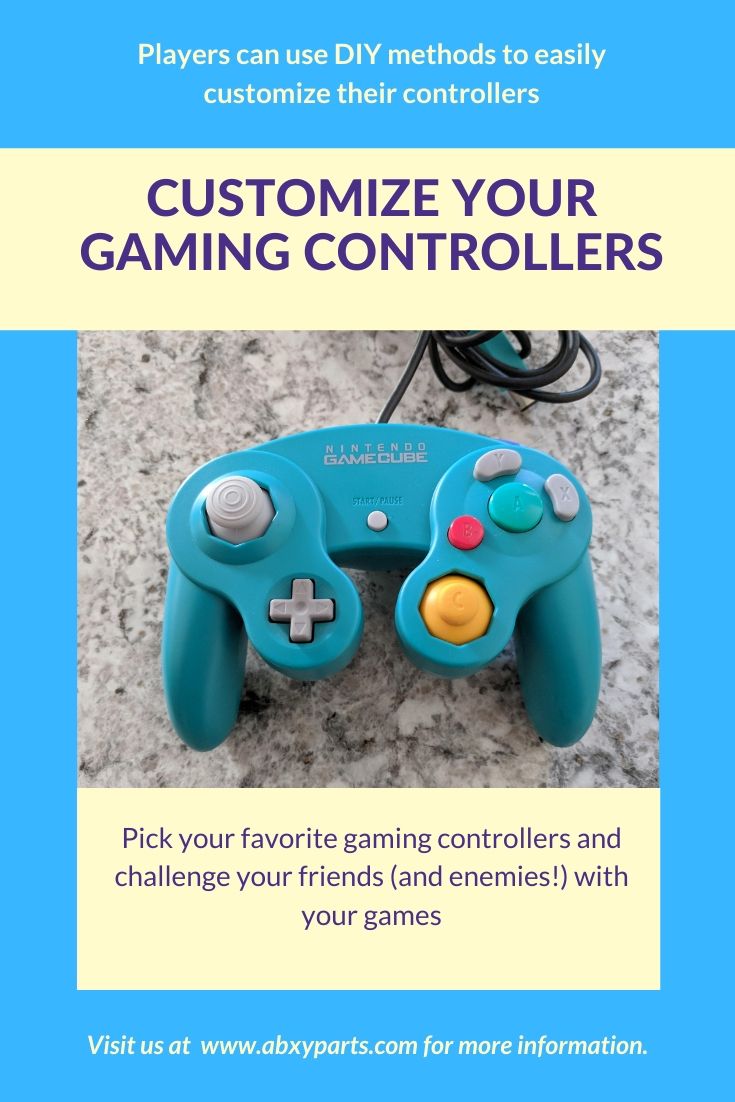This advertisement poster, seemingly photographed indoors, features a vibrant and eye-catching design set against a light blue background. The center of attention is a Nintendo GameCube controller, which rests on a granite countertop. The controller is predominantly light blue with an array of colorful buttons: a yellow button, a red button, a green button, and several gray buttons.

At the top of the poster, bold blue or purple text in a yellow box announces, "Customize your gaming controllers," encouraging players to use DIY methods to easily personalize their controllers. Below the image of the controller, another line of text in the same yellow box invites gamers to, "Pick your favorite gaming controllers and challenge your friends (and enemies) with your games!"

Finishing off the advertisement at the bottom of the image, clear yellow text directs viewers to visit, "www.abxyparts.com for more information," completing this compelling call to action.